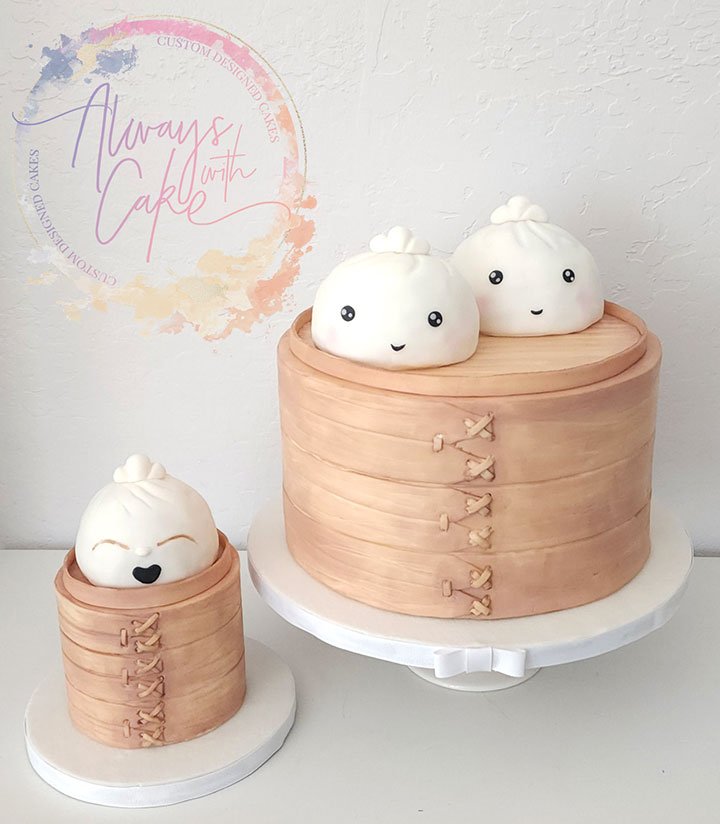The promotional picture for Always with Cake showcases custom-designed cakes that intricately resemble stacked circular sewing boxes made from bamboo. The image, ideal for a cake sales website, features a logo in the upper left-hand corner with cursive text reading "Always with Cake." The logo is encircled with watercolor accents in shades of pink, white, light brown, and blue. The display includes two cakes: a large cake positioned in the upper right area and a smaller one in the lower left, both reminiscent of beige bamboo baskets. Each cake is adorned with charming satchels resembling plump, white cloth buns with cute, smiling faces; one on the small cake appears to be yawning. The cakes are nestled on a sleek white cake stand, emphasizing their intricate and adorable design elements.